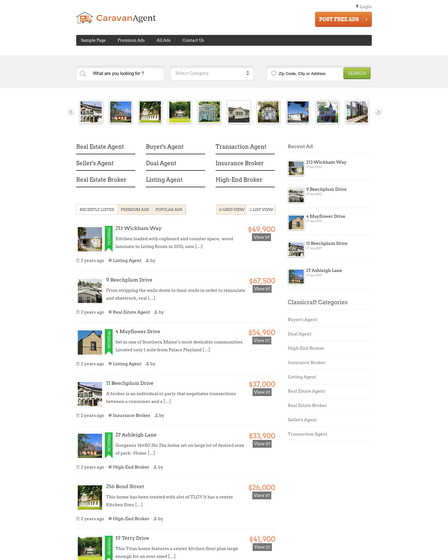The image features a detailed webpage layout for a real estate platform named "Caravan Agent." In the top left corner, the site's name is prominently displayed, while an orange button labeled "Post Free Ads" is positioned on the top right. The page has a black navigation strip containing small, somewhat hard-to-read tabs that appear to be labeled "Premium Ads," "AI Ads," and "Contact Us."

Below the navigation strip, there is a search section with two search bars. The first search bar has a placeholder text that reads, "What are you looking for?" and allows users to refine their search by company. The second search bar prompts for "Zip code, city, or address" and features a green search button.

Beneath this, a row of images showcases various houses, each accompanied by tabs categorizing different types of real estate professionals, including Real Estate Agent, Seller's Agent, Real Estate Broker, Buyer's Agent, Dual Agent, Linking Agent, Transaction Agent, Insurance Broker, and High-End Broker.

Further down, the main section features multiple real estate listings. One prominent listing displays an address, "213 Wickham Way," priced at $49,900. Accompanying this listing are six additional house images, each with associated pricing. Some listings are marked with small green icons or tags. On the right side of the page, smaller, more condensed listings continue, providing additional home options and price details.